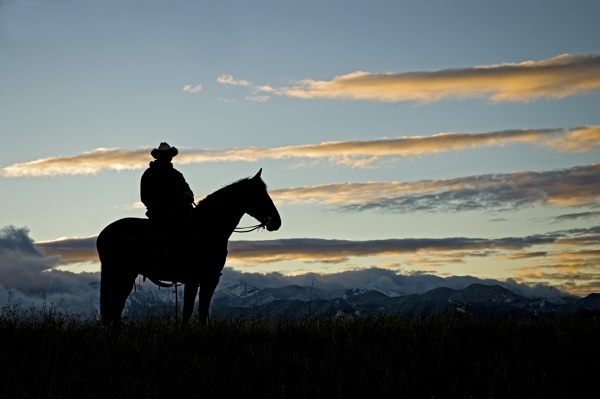In this image, we see a striking, black silhouette of a man on a horse positioned on the left side. The man, donned in a cowboy hat and a thick-looking jacket, is riding a stationary horse. The ground beneath them is dark and shadowy, with faint hints of green grass peeking through at the edges. The backdrop features a distant, grayed-out mountain range. Above the mountains, the sky transitions from a darker to a lighter blue as it nears the horizon, interrupted by streaks of cream-colored clouds. The setting sun casts an orange glow on the edges of these clouds, adding a warm hue to the otherwise cool tones of the scene. The right side of the image prominently features these clouds, while the upper left reveals a clearer expanse of sky.